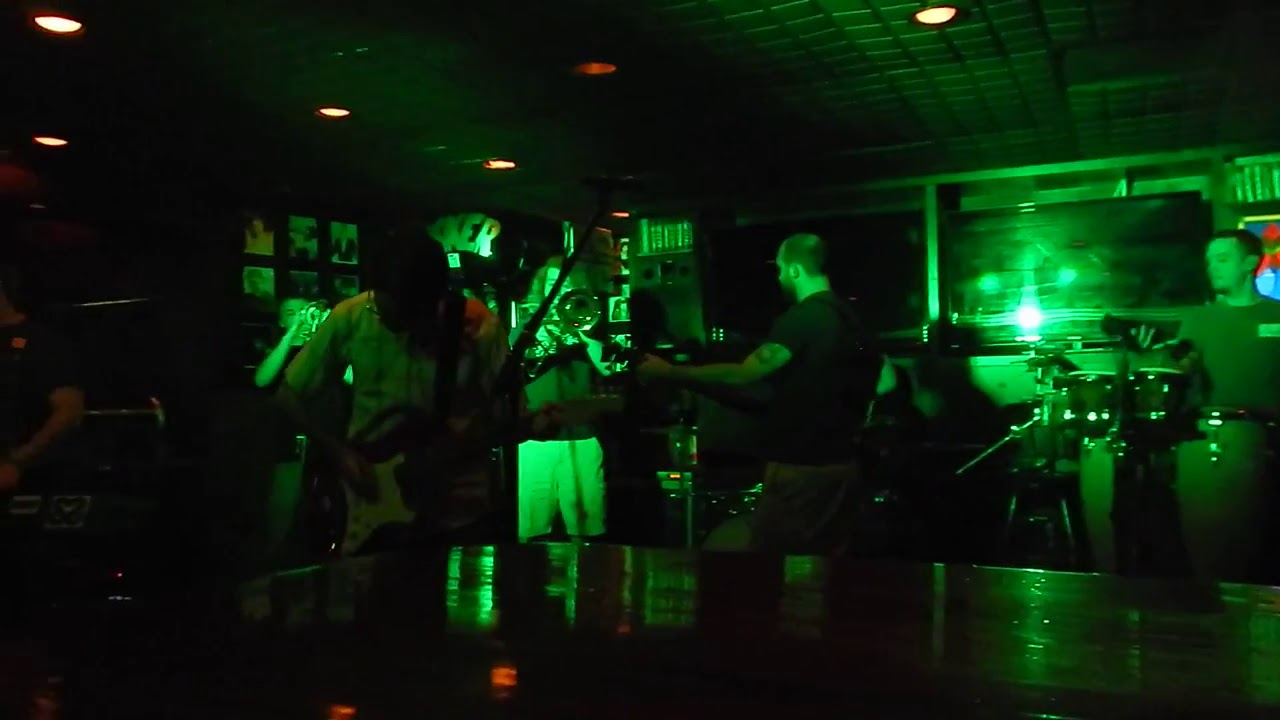This image captures a low-light, green-tinted scene of a band performing in a bar or pub setting. The green lighting bathes the entire room, making the band members and their surroundings glow in an eerie hue. The ceiling, consisting of small square tiles, is dotted with small circular yellow lights that add to the atmospheric ambiance. 

At the forefront, a reflective counter or table surface spans the bottom of the image, hinting that the photo was taken from someone sitting at a wooden table. The band is arranged with several musicians: A guitarist stands mid-frame, looking back at a fellow band member while playing. To the far right, a drummer appears to be using a bongo set. On the left, a bassist is clearly visible. 

Additionally, the band includes brass instruments, with a trombone player and a trumpet player slightly visible on the left side. The overall composition and the eclectic mix of instruments suggest that the band may be playing ska or similar genre. Despite the low quality and dim lighting of the image, the vivid green illumination and the band's lively arrangement make for a striking visual.